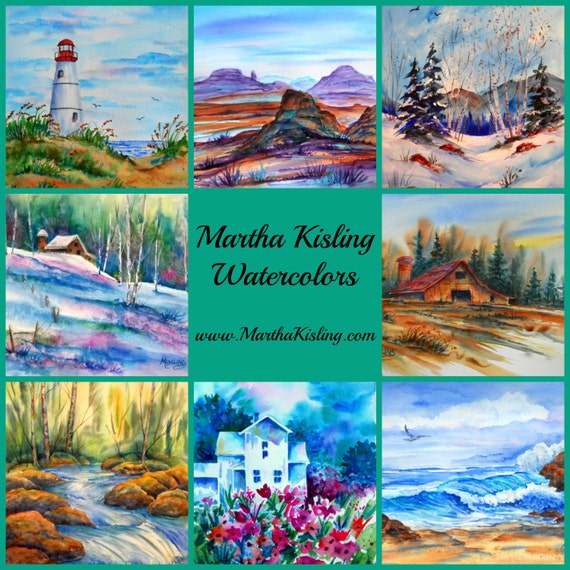The image comprises a 3x3 grid of watercolor paintings by Martha Kisling, with the center square displaying a light green background and the text "Martha Kisling Watercolors" alongside the website "www.marthakisling.com" in black script. Surrounding this central square are eight distinct landscape paintings. 

In the top left, a white-walled, red-topped lighthouse overlooks the ocean. The top middle features a painted desert with multicolored cliffs, purple trees, sandy copper-red stretches, and blue hues. The top right displays a peaceful snow-covered valley with mountain peaks in the background.

On the left center square, there’s another serene snow scene with pines and varied shades of purples and blues. The right center shows a quaint farmhouse amidst fields of snow. The bottom left depicts a rocky mountain stream. The bottom middle showcases a white house set against a backdrop of vibrant flower gardens. Lastly, the bottom right captures an ocean beach with crashing blue waves. The collection of images reflects the artist’s diverse exploration of nature, rendered in a soft, watercolor style.